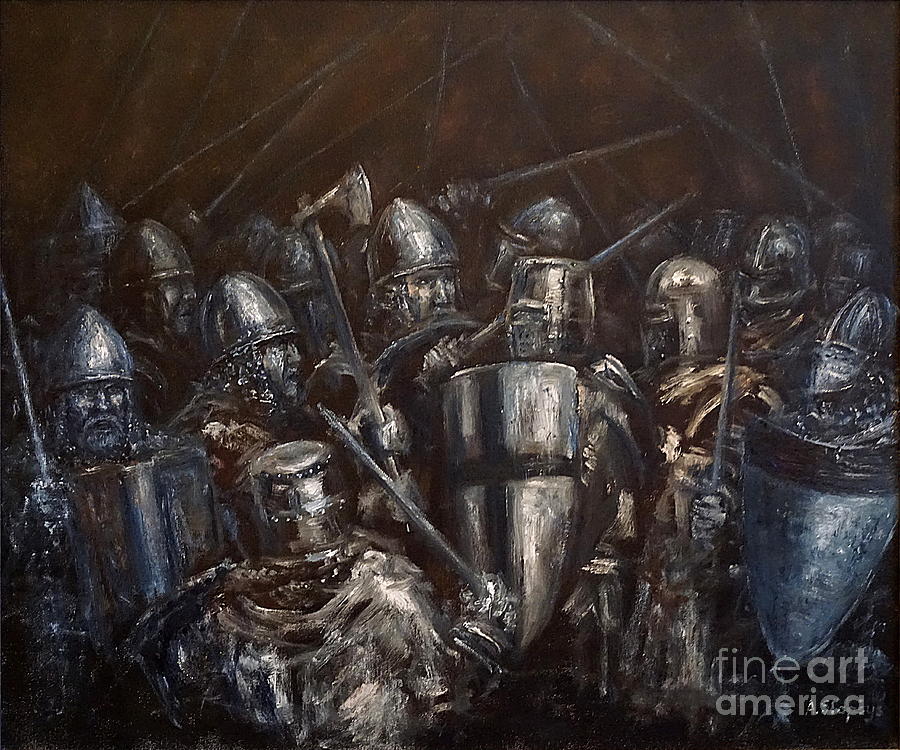This is a dark, impressionistic-style oil painting depicting a large group of men, estimated to be between 15 to 20, clad in medieval-inspired armor preparing for battle. The textures are heavy, with prominent black, blue, and gray tones underlining the somber mood of the scene. Some of the men appear to be Vikings, identifiable by their pointed helmets and rudimentary weapons such as swords, spears, and a hatchet. A standout feature is a shield adorned with a black cross, prominently carried by one of the central figures. The image also includes soldiers with dark gray helmets and bright silver shields, adding to the chaotic energy present. Many of the soldiers wear helmets that obscure their faces, contributing an anonymous and intense feel to the gathering. The bottom right corner of the painting bears a white watermark reading “Fine Art America,” underscoring its origins as fan art.